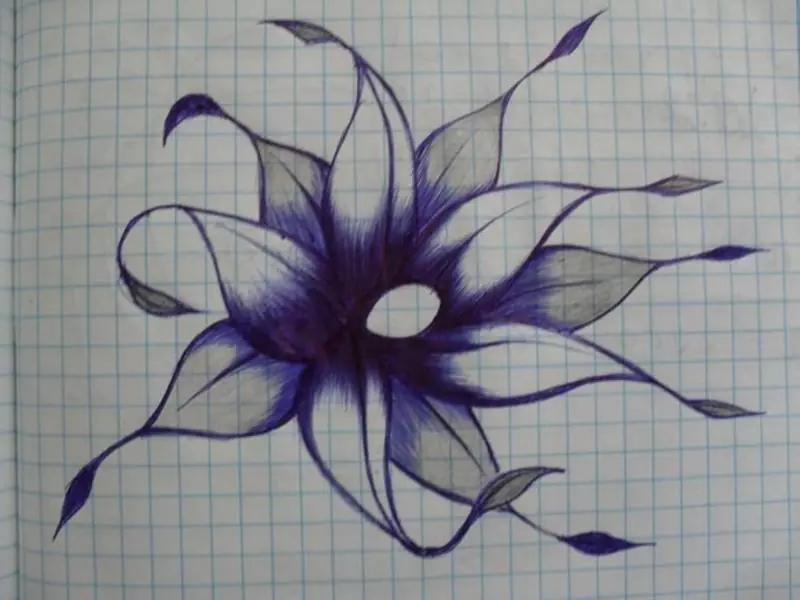This image features an intricate ink drawing of a flower on blue graph paper, characterized by its detailed lines and shading. The flower boasts an eye-catching center, depicted as a clear, white circle that reveals the squares of the graph paper underneath. Radiating from the center are six large petals, shaded with dark blue ink that gradually fades towards the edges, blending into white. These primary petals have long, flowing, leaf-like shapes with pointed, diamond-shaped extensions at their tips. Surrounding these main petals, there are additional layers: three green petals and a set of five secondary petals shaded in light gray, possibly done with a pencil. The overall arrangement gives the flower a complex and layered appearance, accentuated by the ink's blackish-purple hue, making the design both detailed and visually captivating.